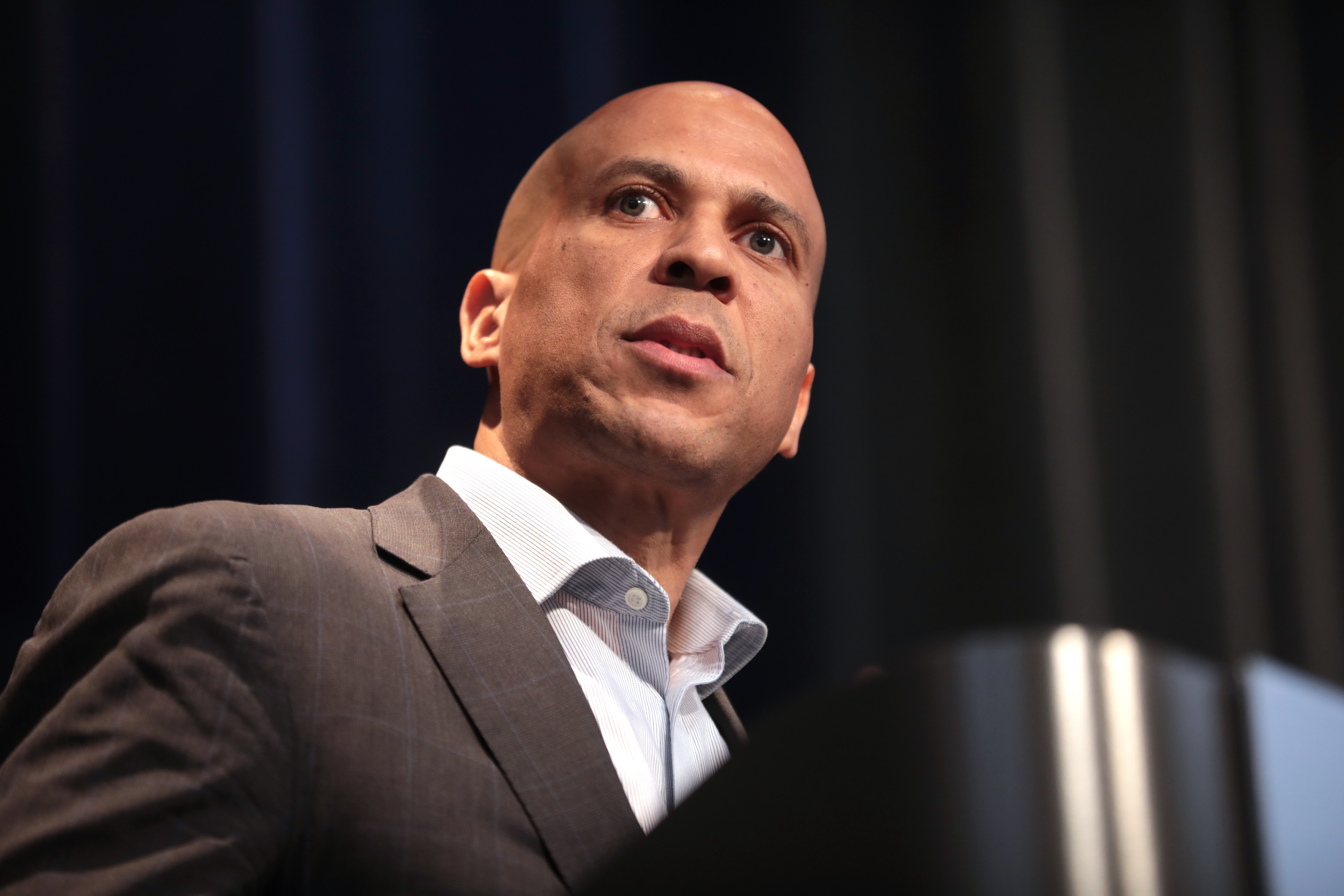The photograph features an African American man, clean-shaven and bald, wearing a black suit paired with a white dress shirt. He stands at a podium, slightly positioned towards the center of the image. His long-legged stature and left-handed disposition are noticeable, and he is facing towards the right-hand side, his body angled in a 5 o'clock direction while his eyes glance upwards to the 7 o'clock position. His facial expression reflects a mix of confusion and slight surprise, his chin directly pointed towards the camera. The background is a dark, blurred expanse, transitioning from black to blue hues, with details suggesting black curtains. A blurred corner of the podium is visible in the lower right part of the image. The setting is indoors, possibly during a speech or public address, with the overall scene devoid of any text but rich in varying shades of gray, blue, and black.